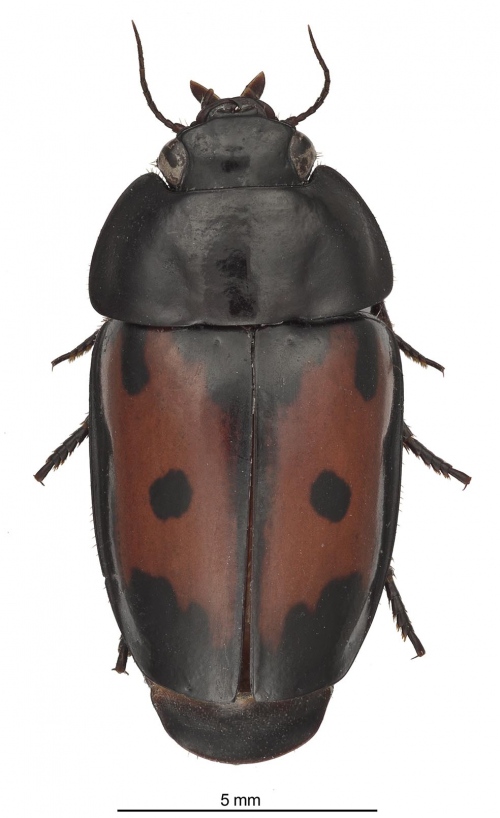This image displays a close-up view of a beetle with a body length of approximately five millimeters, as indicated by the scale at the bottom. The beetle's body features a hard, smooth, and almost shell-like exoskeleton. The head is entirely black, equipped with two prominent eyes on either side, a pair of antennas, and two small pinchers. The beetle has six legs, three on each side, that are short and fuzzy, adding a textured appearance. Its upper body and head are predominantly black, transitioning to a dark, rust-colored red for the wings, which are marked with black spots. The photo, taken from an overhead perspective, highlights the beetle's detailed and intricate anatomy.